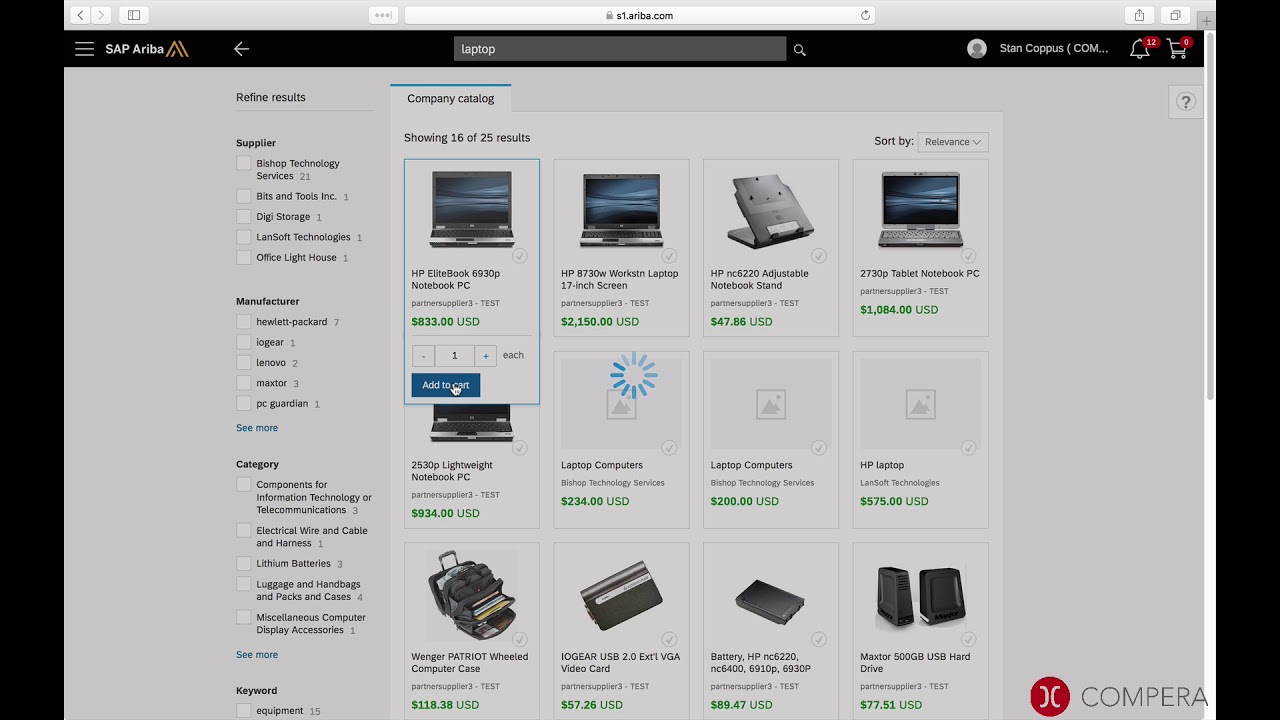Screenshot of a SAP Ariba webpage featuring a gray and white color scheme with black accents. At the top of the page, it prominently displays the SAP Ariba logo, including a yellow "A" graphic. There is a search bar with a locked icon, indicating it is set to Ariba.com, and within the search bar, the user has entered the query "laptop". An arrow pointing left is present next to the search bar. The interface shows white font on a gray background. A notification icon is lit up with 12 alerts, and there's a shopping cart icon to the right, showing one item placed in it. Various product options are displayed, including an HP notebook priced at $833, another HP laptop with a 17-inch screen listed for $2150, and a notebook priced at $1084. Additionally, the page shows several accessories available for purchase.